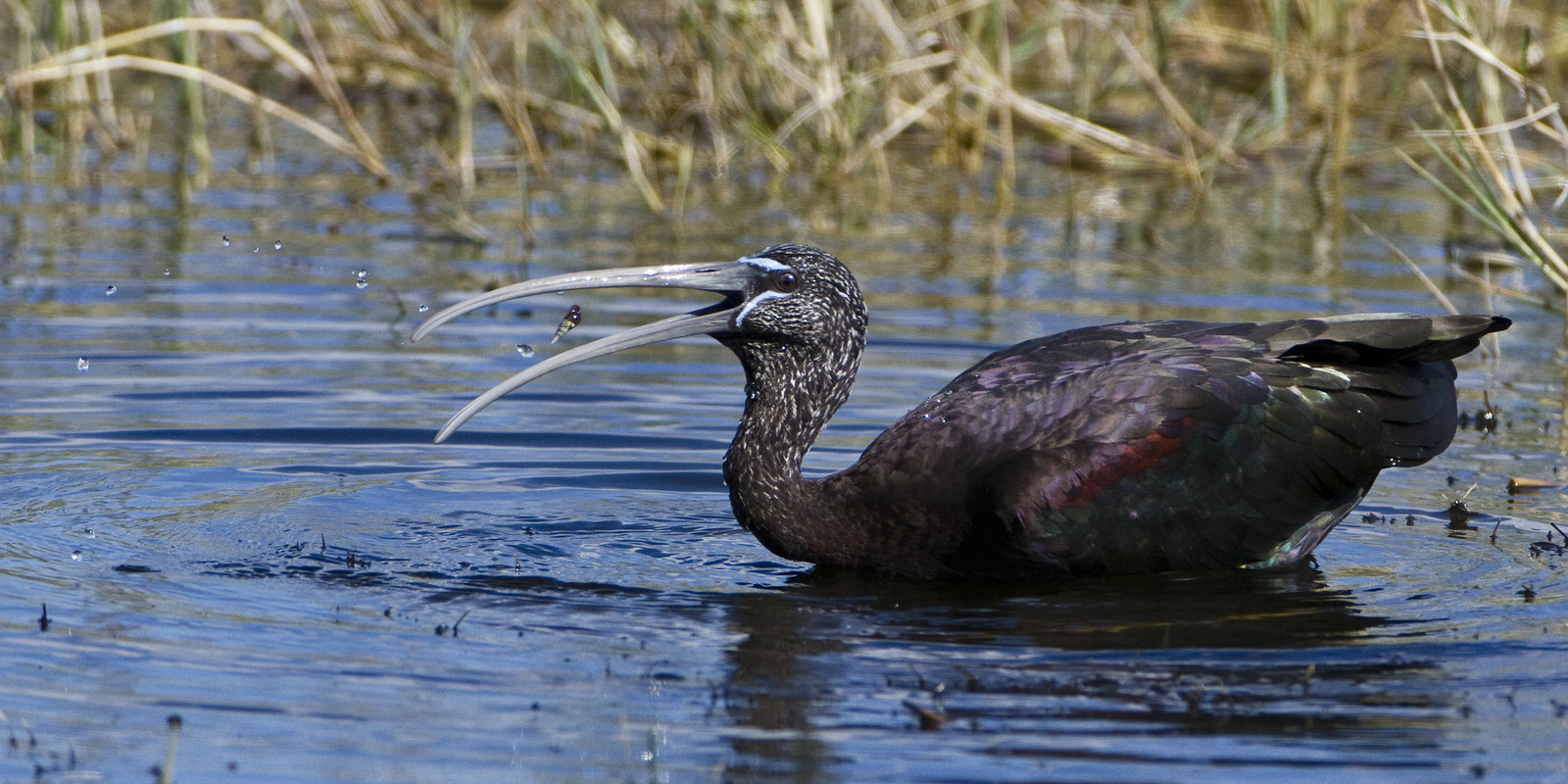In this outdoor image set in a marshland, a large bird resembling a duck with a notably long, slightly curved beak is depicted in the water, facing left. The bird's color is predominantly brown on the head and neck, enhanced with patches of white, especially around the eye and lower cheek. Its body showcases a mosaic of dark feathers with hints of purple and black, and subtle touches of red on the wings. The bird's long, off-white beak is slightly open, capturing another bird within it, highlighting its carnivorous nature. The clear water beneath it ripples from the bird's movements, while the background is adorned with reeds, cattails, and other marsh vegetation at varying stages of life, indicating a rich, natural habitat.